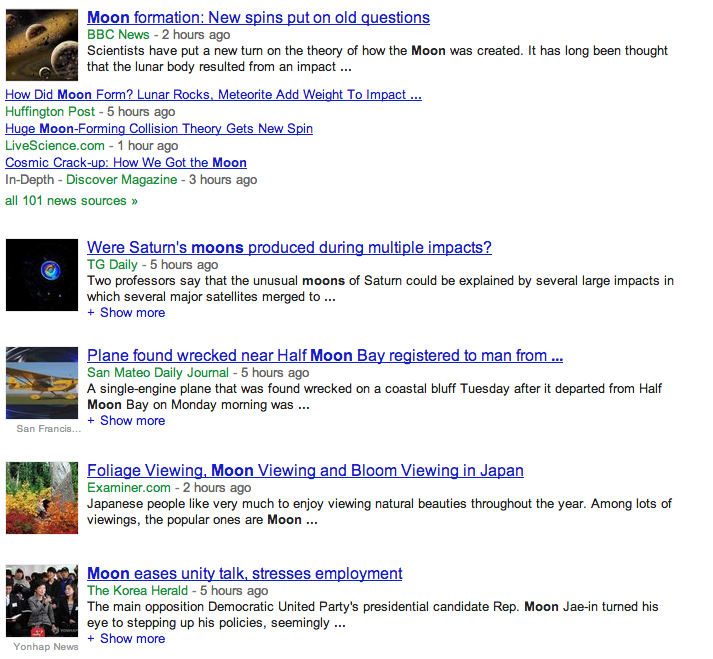The image is a screenshot of search results related to recent discoveries and theories in lunar and space science. In the top left corner, there is a photograph of space featuring planets. To the right of the image, the headline in blue reads, "Moon formation: New spins put on old questions - BBC News, two hours ago." The article discusses a fresh perspective on the long-held theory that the Moon was created from a massive impact.

Below this, another headline states, "How did the Moon form? Lunar rocks, meteorites add weight to impact theory - Huffington Post, five hours ago." This is followed by "Huge Moon-forming collision theory gets new spin - Live Science, one hour ago," and "Cosmic crack-up: How we got the Moon - an in-depth piece by Discover Magazine, three hours ago." There is an option to view all 101 related news sources by clicking a right arrow.

Further down, there's a section with a photograph and a headline, "Were Saturn's moons produced during multiple impacts? - TG Daily, five hours ago." The article explores a theory by two professors proposing that the unusual moons of Saturn could have resulted from several impacts where multiple satellites merged.

At the bottom of the search results is a news brief saying, "Plane found wrecked near Half Moon Bay, registered to a man from... - San Mateo Daily Journal, five hours ago." The report details how a single-engine airplane was found wrecked on a coastal bluff after departing Half Moon Bay on Monday morning. There is an option to "show more" for additional details on both the Saturn moons and the airplane wreckage.